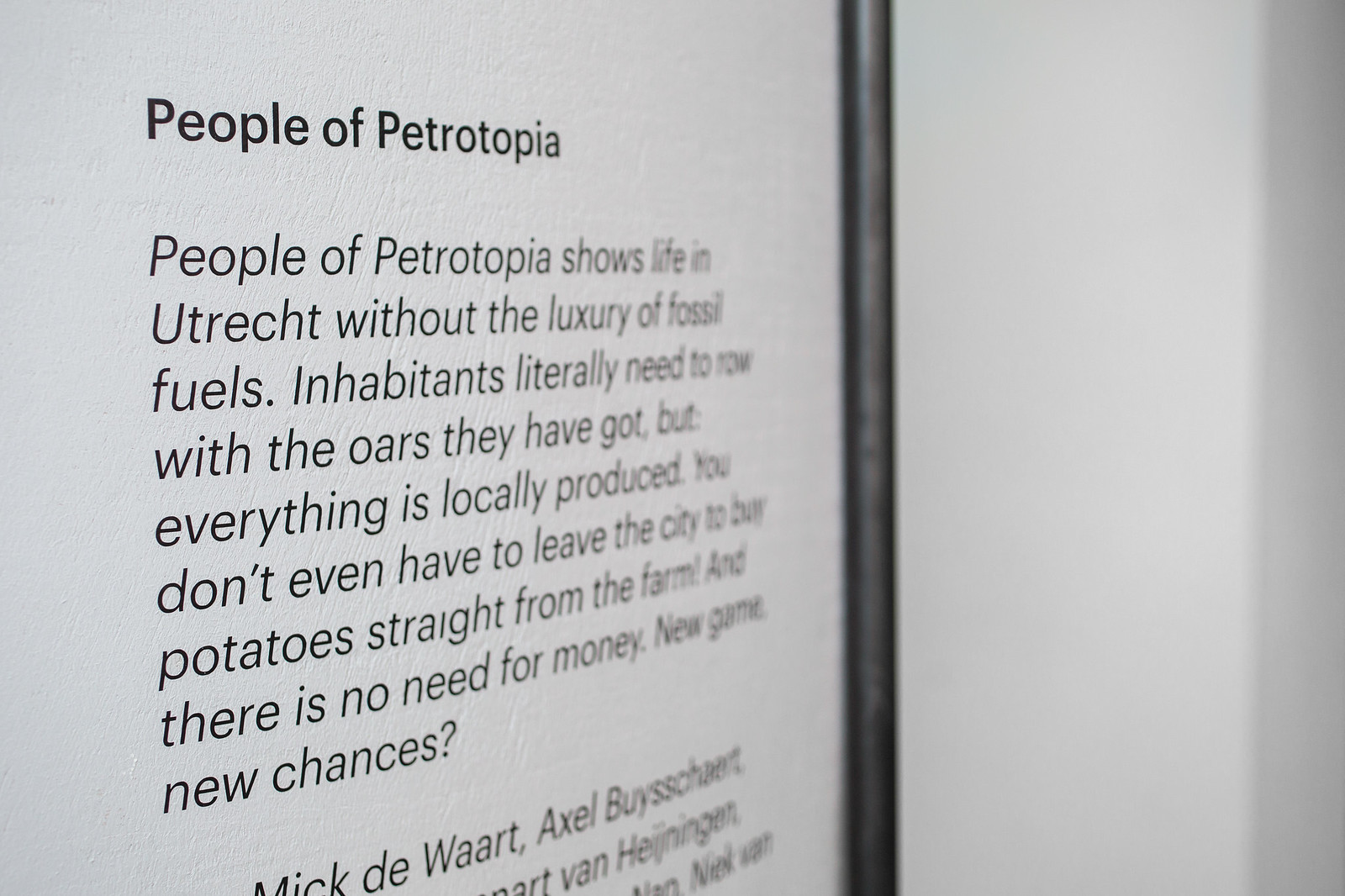This detailed photograph captures a close-up of a text panel, possibly from a museum exhibit. The panel is a horizontal rectangular shape with a white background and black text arranged horizontally in rows. The title at the top reads "People of Petrotopia." Below, a paragraph describes life in Utrecht without the use of fossil fuels: “People of Petrotopia shows life in Utrecht without the luxury of fossil fuels. Inhabitants literally need to row with the oars they have got, but everything is locally produced. You don't even have to leave the city to buy potatoes straight from the farm, and there is no need for money. New game, new chances.” Towards the right side of the panel, a thin vertical black rectangle runs from top to bottom, resembling the center binding of a book. Adjacent to this separator, on the right side, is a blank page. Below the paragraph, names are partially visible: Mick DeWart, Axel Bouchart, and others like Van Hingen and Van Nielsen, although some are cut off. The overall image is taken at an angle with a metal frame or bar visible in the foreground.